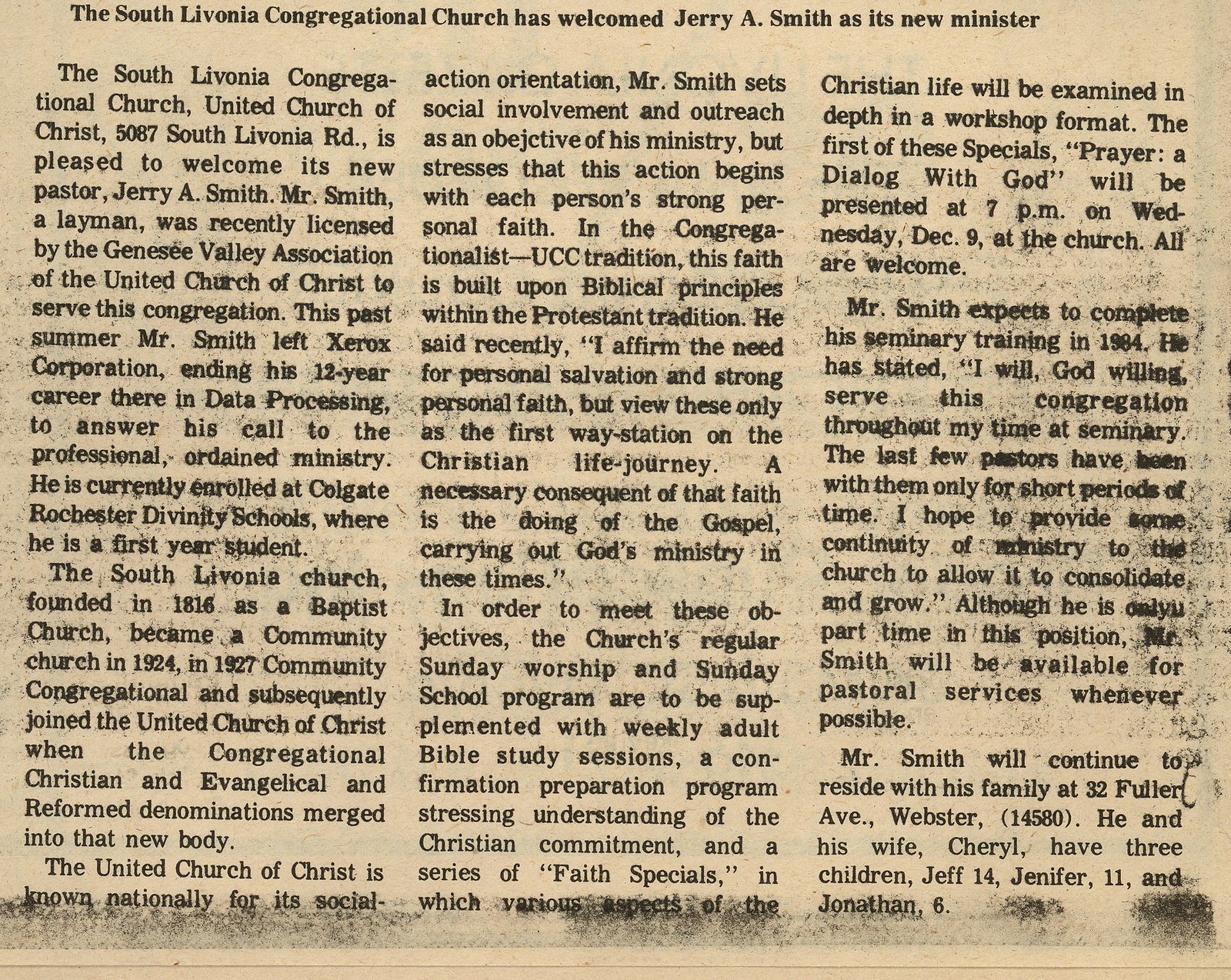This newspaper article announces the appointment of Jerry A. Smith as the new minister of the South Livonia Congregational Church, United Church of Christ, located at 5087 South Livonia Road. The article details how Mr. Smith, a recently licensed layman by the Genesee Valley Association of the United Church of Christ, left a 12-year career in data processing at Xerox Corporation to pursue his calling to the ordained ministry. He is a first-year student at Colgate Rochester Divinity School and aims to complete his seminary training by 1984.

Mr. Smith emphasizes the importance of social involvement and outreach stemming from strong personal faith, resonating with the United Church of Christ's tradition of social action. He articulates his mission to support the congregation in growing deeper personal faith that translates into active gospel ministry. The church plans to complement its regular worship and Sunday school program with weekly adult Bible study sessions, a confirmation preparation program, and a series of in-depth faith workshops, starting with "Prayer: A Dialogue with God" at 7 p.m. on Wednesday. 

Mr. Smith resides with his wife, Cheryl, and their three children, Jeff, 14; Jennifer, 11; and Jonathan, 6, at 32 Fuller Avenue, Webster, NY, 14580. He expresses his commitment to providing continuity of ministry, hoping to stabilize and foster growth within the congregation during his tenure.